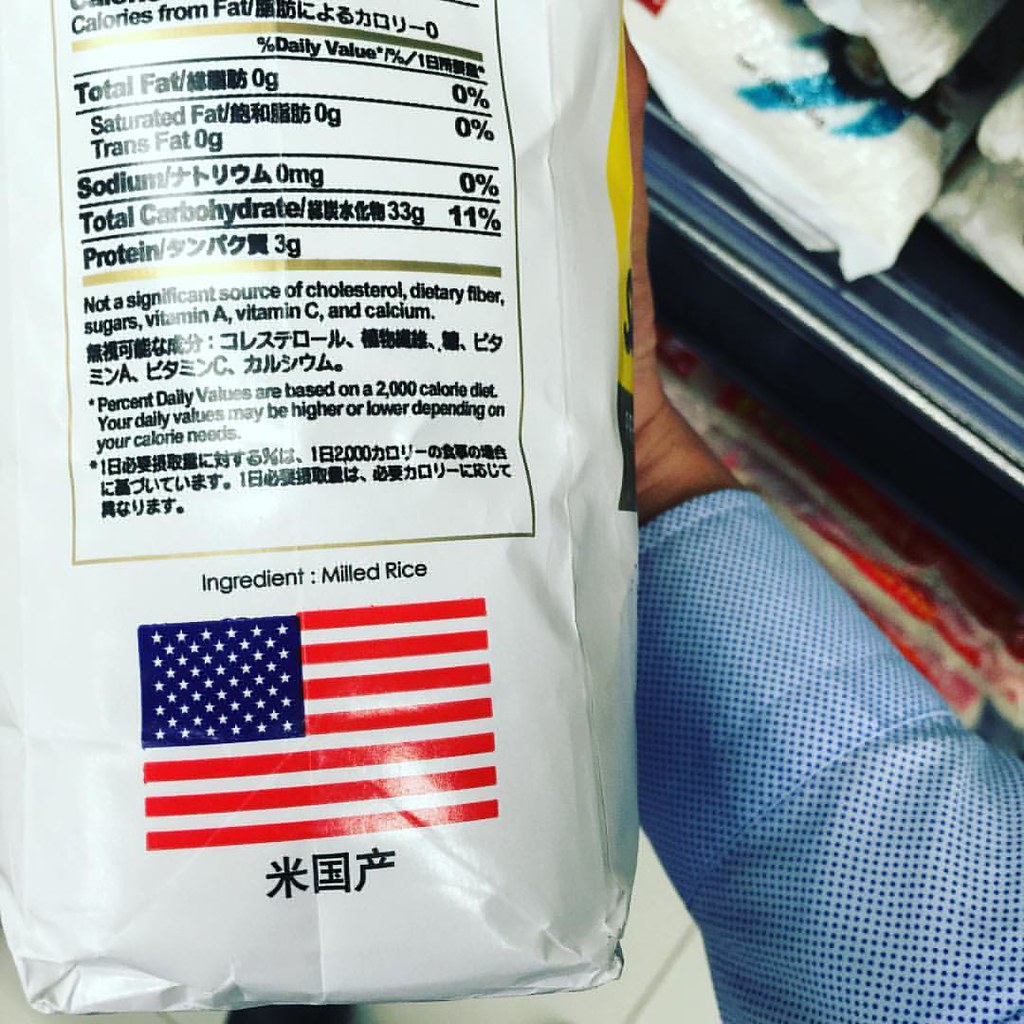A man in a long-sleeve shirt is prominently featured in the image, facing the camera. He holds a bag with the nutritional information panel displayed clearly. The bag, likely pulled from a nearby display—which may or may not be refrigerated—contains milled rice. It showcases both English and Asian writing, indicating an international product. The American flag is visible at the bottom of the packaging, hinting at its distribution or marketing origin. The upper part of the bag is slightly cut off, but crucial nutritional details such as total fat, sodium, total carbohydrates, and protein are legible, alongside their Asian counterparts. Red items can be seen on the floor beneath the display, adding a splash of color to the setting.